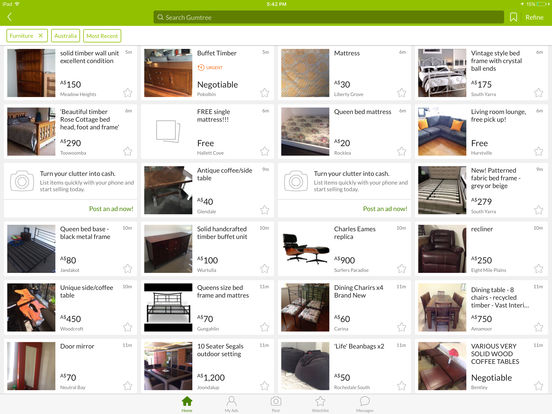The image features a light green border at the very top, adorned with tiny text centered, on the top right, and the top left, all too small to decipher. Beneath the border is a dark green search bar, followed by a white background that dominates the lower section of the image. There are three clickable buttons prominently displayed below the search bar, with one of the buttons labeled "Furniture"; the labels on the other two buttons are unreadable.

Further down, the image is divided into four rows, each containing six rectangular sections showcasing various items for sale. Each section includes a picture of the item on the left, accompanied by a description and price details. On the right side of each section, a star icon is visible. Scanning through the prices, the top-left corner features items listed at 150, 290, 80, 450, and 70 units of currency.

Further information includes ambiguous text with assorted pricing and details, which reads "negotiable," "free," and prices such as 40 and 100 units. Much of the additional text is blurred and illegible, rendering further details unclear.